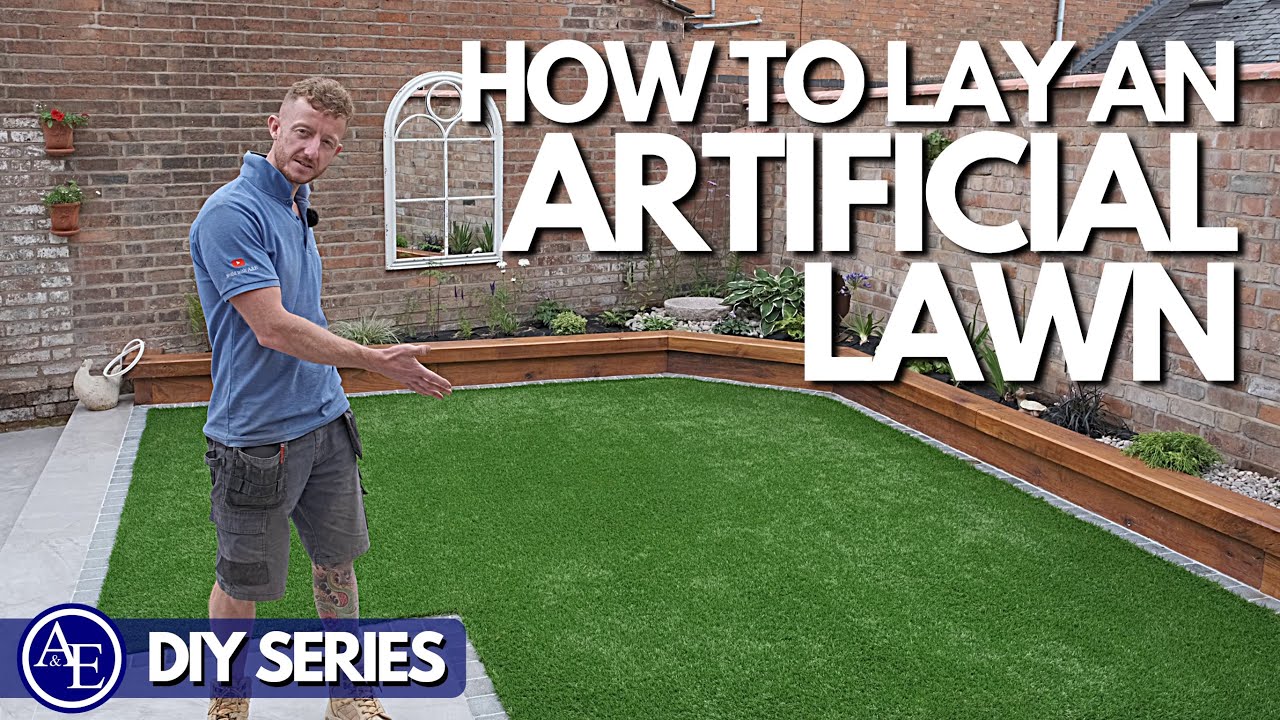In a tranquil backyard setting, a Caucasian man in his mid-30s to 40s stands on an impeccably green, artificial lawn. He is wearing a blue polo t-shirt, dark gray cargo shorts, and shoes, boots, or sneakers. His short, reddish-blonde hair and leg tattoos are visible. The lush lawn, which looks freshly mowed, extends across the space, bordered by brick walls adorned with flower pots and a landscaped wooden flower bed filled with various plants.

The background reveals the exterior of a house with brick walls, adding a cozy touch to the scene. Additional elements such as a vase, a water feature, and what might be a football helmet contribute to the peaceful ambiance. The scene, dominated by shades of green, gray, and white, exudes a sense of tranquility and outdoor relaxation.

The man is gesturing toward the artificial lawn, proudly showing off his work, while the image prominently features branding for the A&E DIY series. Positioned in the top right corner, white letters announce the topic: "How to Lay an Artificial Lawn." This image serves as an engaging header for a website, demonstrating the man's expertise and connection to the A&E DIY series.